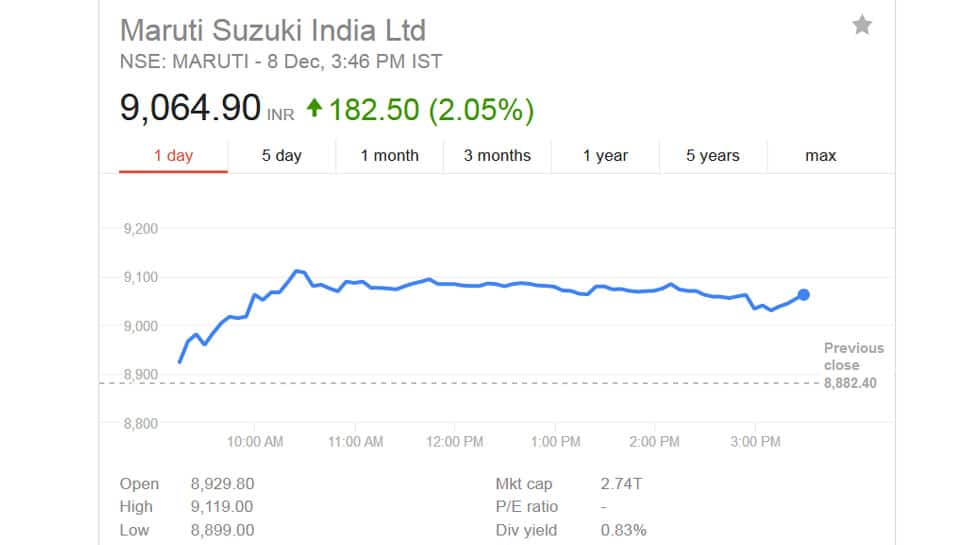Screenshot of a Graph Displaying Stock Performance of Maruti Suzuki India LTD

This image showcases a detailed bar graph depicting the stock performance of Maruti Suzuki India LTD, listed on the NSE (New York Stock Exchange). The graph is dated 8th December and was captured at 3:46 PM IST. The current stock price is prominently displayed at the top in bold black numbers as ₹9,064.90 INR. Below it, in green digits with an upward arrow, the stock shows an increase of ₹182.50 (2.05%).

The bar graph provides various time frame options including '1 Day' (highlighted in red), '5 Day', '1 Month', '3 Months', '1 Year', '5 Years', and 'Max'. The Y-axis of the graph ranges from 8,800 to 9,200, indicating small incremental changes, while the graph itself shows fluctuations in stock price between slightly above ₹8,900 and just below ₹9,000.

Below the graph, key statistics of the stock are listed:

- **Open:** ₹8,929.80
- **High:** ₹9,119.00
- **Low:** ₹8,899.00
- **Market Cap:** 2.74T
- **P/E Ratio:** (not provided)
- **Yield:** 0.83%

Overall, this screenshot provides a comprehensive overview of the recent stock performance of Maruti Suzuki India LTD on the NSE.